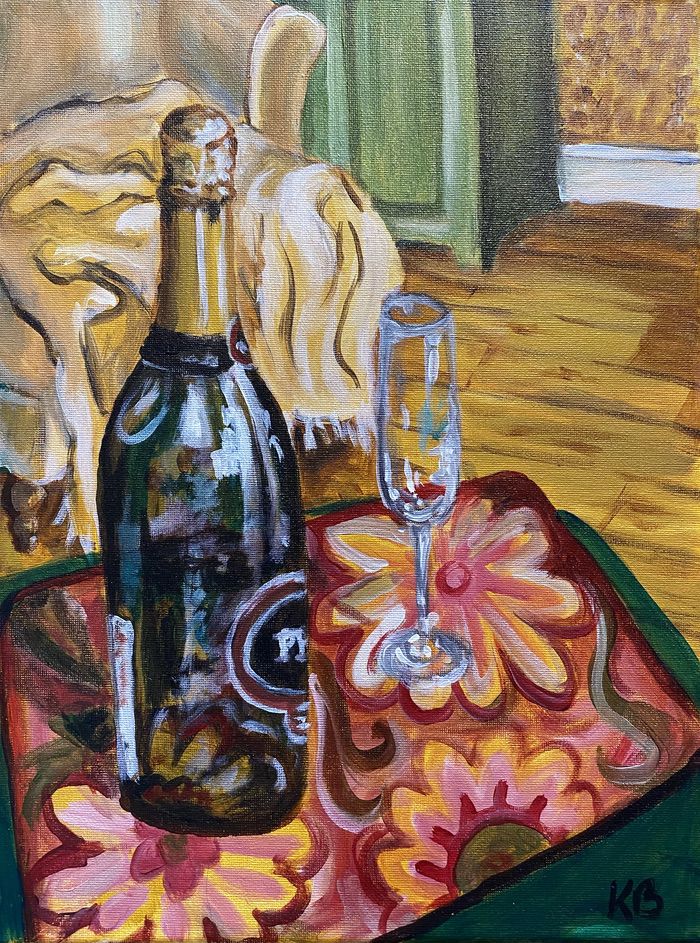This oil on canvas painting captures a detailed still life scene with a vibrant, impressionistic touch. Central to the composition is a green tray adorned with painted flowers in shades of yellow, pink, and red. Resting on the tray is a greenish wine or champagne bottle, showcased in a side view with a gold cap and neck, and a black label with faint white lettering and a red frame. Accompanying the bottle is a clear, flute-like champagne glass. The setting includes a light-colored wooden floor, and in the background, a green piece of furniture—possibly a cabinet or shelf—stands against a brown wall with a white baseboard. Additionally, there is a partial glimpse of a white armchair draped with a yellow blanket. The bottle bears the partially readable initials "P" and possibly "Y," and the artist’s signature is identified by the initials "KB." The overall style leans towards impressionism, eschewing hyper-realism for a more textured and expressive portrayal.